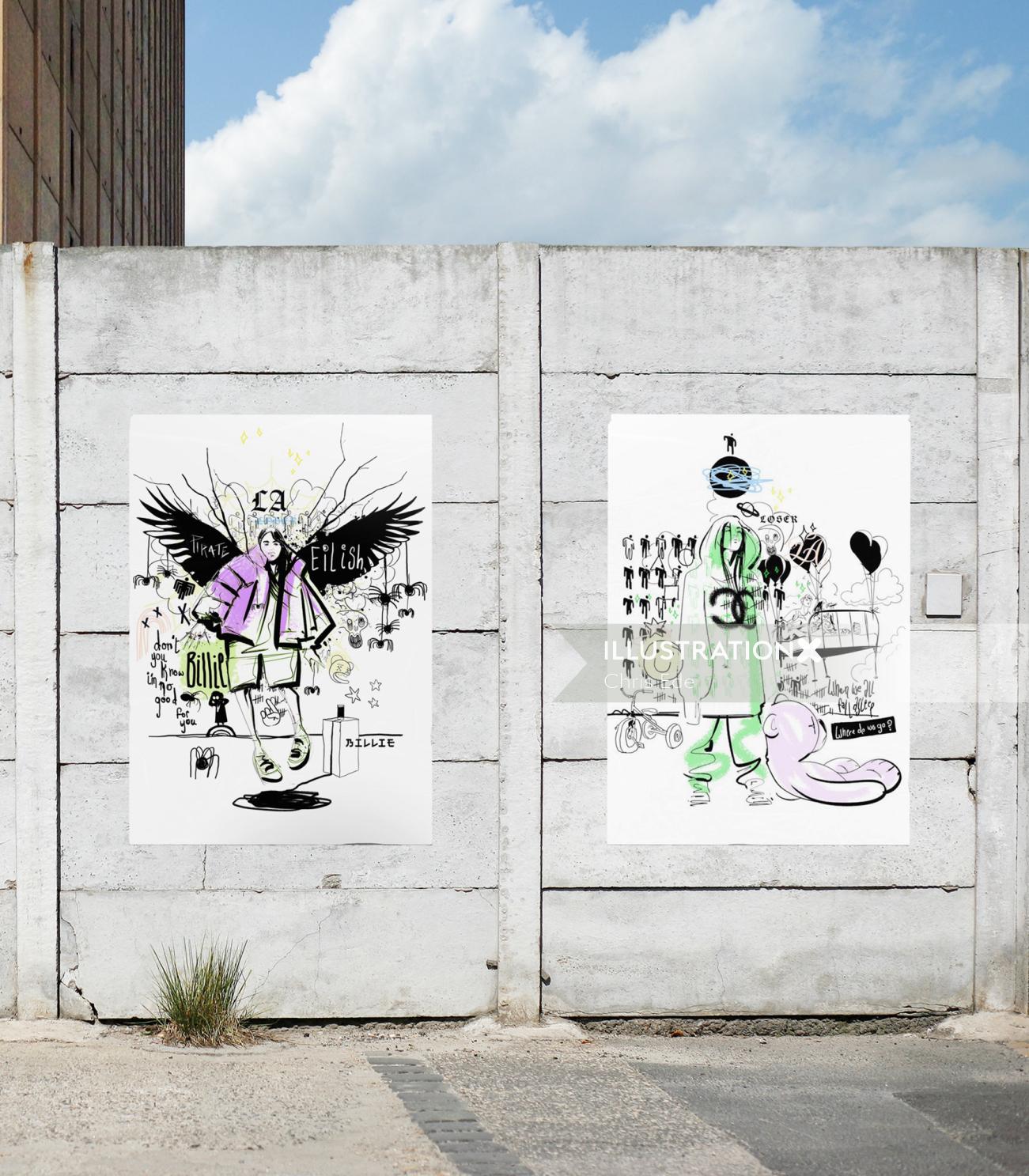In this outdoor scene, a dingy brownish-tan building is partially visible in the top left-hand corner against a backdrop of a blue, cloud-strewn sky. A solid gray fence stretches across the image's background, with a small green weed growing in front of it, separating it from the pavement. Mounted on the fence are two illustrative posters placed side-by-side. The left poster, imbued with purples and whites, depicts a girl with wings adorned with spiderwebs, surrounded by various words. The right poster features a hooded figure in green and blue hues, likely representing Billie Eilish, with the iconic double C's from Chanel visible on the hoodie. A teddy bear is seen lying at the figure’s feet, adding depth to the scene. The area appears to be near a driveway or parking lot, enhancing the urban setting of the artwork.